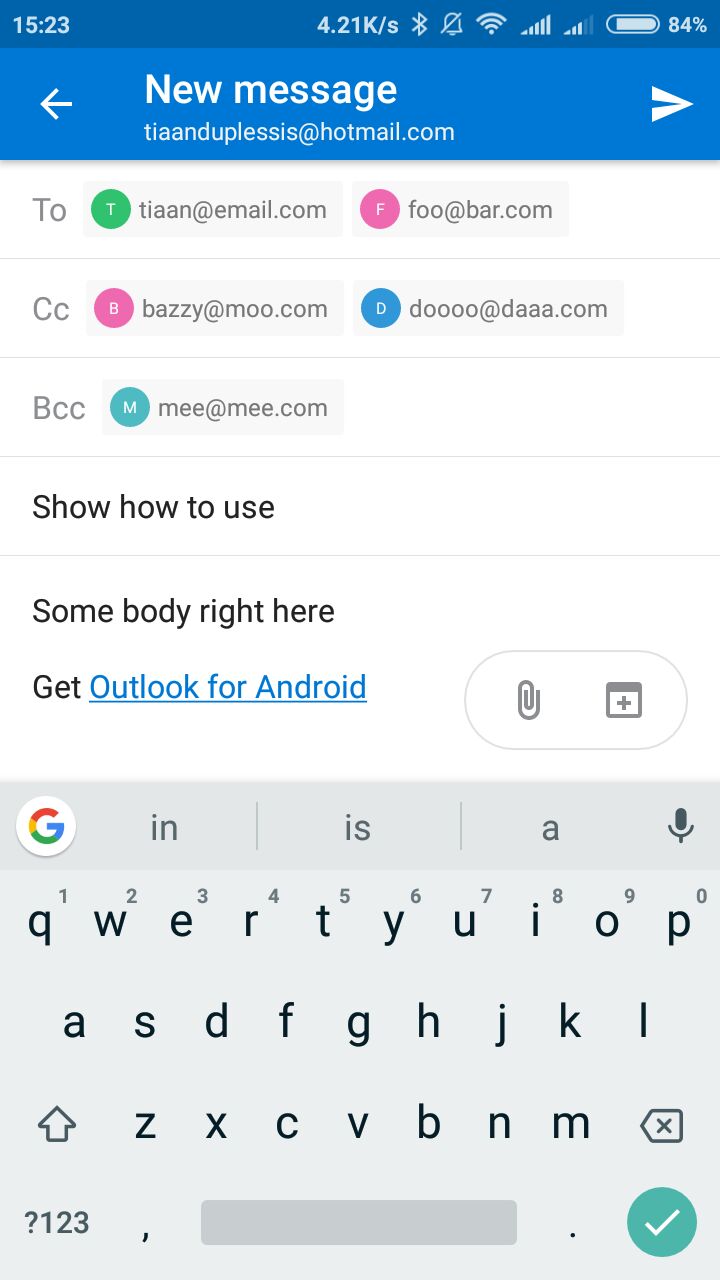This is a detailed screenshot from a person's cell phone. At the very top of the image, there is a thin dark blue border displaying the time "15:23," a speed indicator "4.21K/S," and an assortment of status icons: a Bluetooth symbol, a bell icon with a strike-through indicating the phone is on silent mode, Wi-Fi signal strength, cellular network coverage, and an 84% battery life indicator.

Beneath this, a lighter blue banner reads "New Message." The recipient list includes multiple email addresses: TiaandAblesis at Hotmail.com, Tiaan at Email.com, FOO at BAR.com, CCBAZZY at MOO.com, DOOOO at DAAA.com, and BCCMEE at MEE.com. There is also a prompt to "Show How to Use," followed by the text "Some Body right here" and a suggestion to "Get Outlook for Android."

Also visible are icons for attaching a file, represented by a paperclip, and adding more content, shown as a square outlined in gray with a plus sign in the center. The lower portion of the screenshot displays the phone's keyboard in traditional QWERTY layout. At the top of the keyboard, within the Google suggestion strip, appear the suggestions "IN," "IS," and "A," accompanied by the microphone icon for voice input.